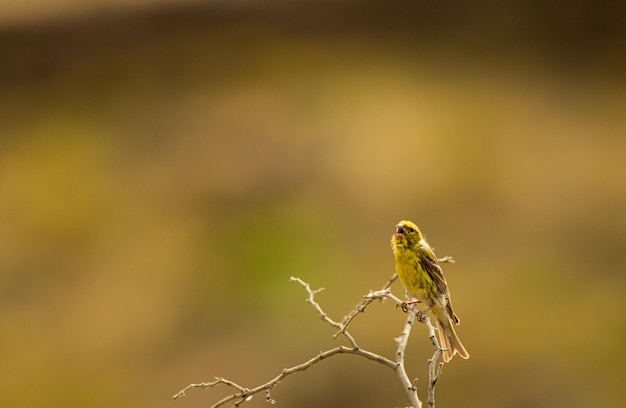This horizontal nature photograph captures a vividly detailed scene where a small Western Serin bird is the focal point. Perched on a thin, almost pale or off-white tree limb, which branches out into several smaller twigs, the bird dominates the lower right section of the image. The branch itself lacks leaves, flowers, or buds. The bird, likely young or molting, displays a bright yellow breast and head with some loose downy feathers sticking out. Its wings are darker, mingling shades of brown, black, and a bit of white, while its tail feathers are gray. The bird's beak is open, possibly indicating it is calling or waiting to be fed. The background is artistically blurred, awash with an amalgam of green, yellow, brown, black, and a hint of purple, enhancing the sharpness of the bird and branch in the foreground. The composition lends a serene, yet dynamically focused glimpse into this moment of avian life in California.